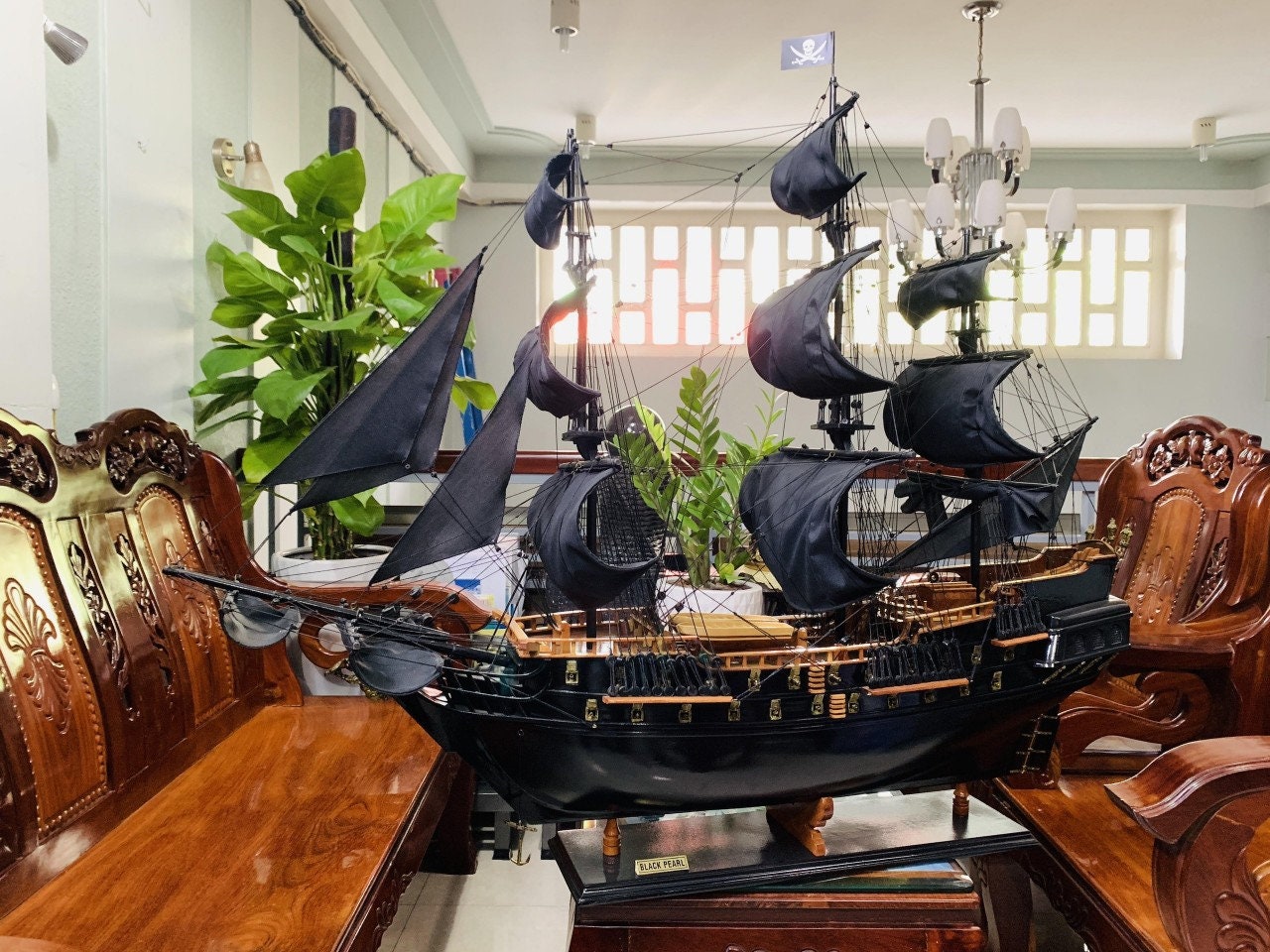The indoor photograph, taken during the daytime, captures a meticulously crafted model of the Black Pearl from the Pirates of the Caribbean movies, prominently displayed on a wooden stand. The ship, approximately three to four feet in length, boasts striking black sails and black-painted hull with light brown accents. A pirate flag adorns its top. The model rests atop a dark mahogany table, which is part of a set that includes a bench to the left and chairs to the right, all finely polished and intricately carved with ornate designs. The room features soft grey walls with white trim and a window with divided panes that lets in natural light. The windowsill is a light tan color. Potted plants in white pots add a touch of greenery to the luxurious setting. In the background, the white walls further emphasize the elegant ambiance of the room, suggesting it might be a private collection or an exhibit in a lavish setting.